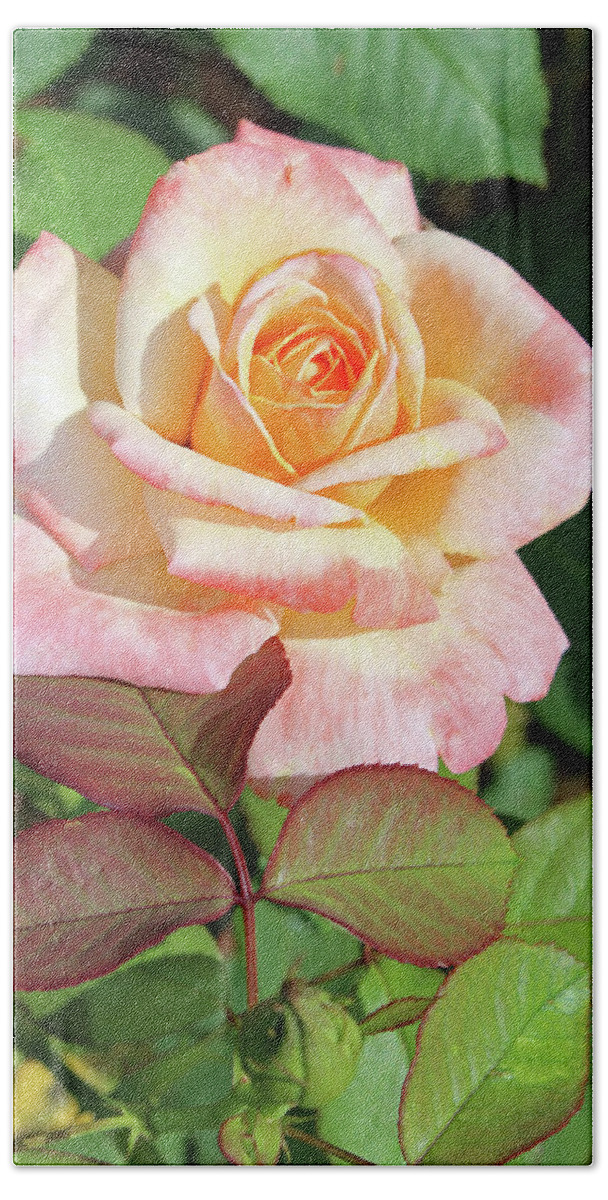The image showcases a close-up digital photograph of a rose, meticulously printed on a sheet of metal for display purposes. The vertically oriented portrait, in a 9 by 16 ratio, features the main subject—a partially bloomed white rose with pink-tipped petals—centrally positioned at the top. This rose is surrounded by a contrasting series of green leaves and vines, enhancing its delicate beauty. A second, much smaller rosebud, still green, can be observed among the foliage below the larger bloom. The intricate detailing of the pink-edged white petals and the vibrant green and partially red leaves beneath make the floral composition visually captivating.